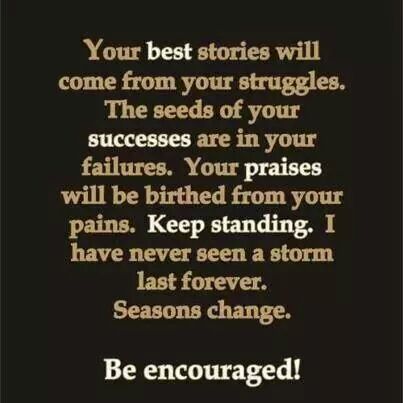The image features a motivational quote displayed centrally on a solid black background. The text is slightly blurry and appears in a mix of khaki-colored and lighter beige letters, giving a goldish and ivory tint effect. The message reads: "Your best stories will come from your struggles. The seeds of your successes are in your failures. Your praises will be birthed from your pains. Keep standing. I have never seen a storm last forever. Seasons change. Be encouraged!" The emphasized words, "best," "successes," "praises," "keep standing," and "be encouraged," are highlighted in a lighter beige color, making them stand out against the rest of the text. The phrase "Be encouraged!" is particularly notable for its emphasis with an exclamation point and its positioning at the bottom of the image. The overall feel is reminiscent of something you'd see shared on social media platforms like Facebook or Instagram.